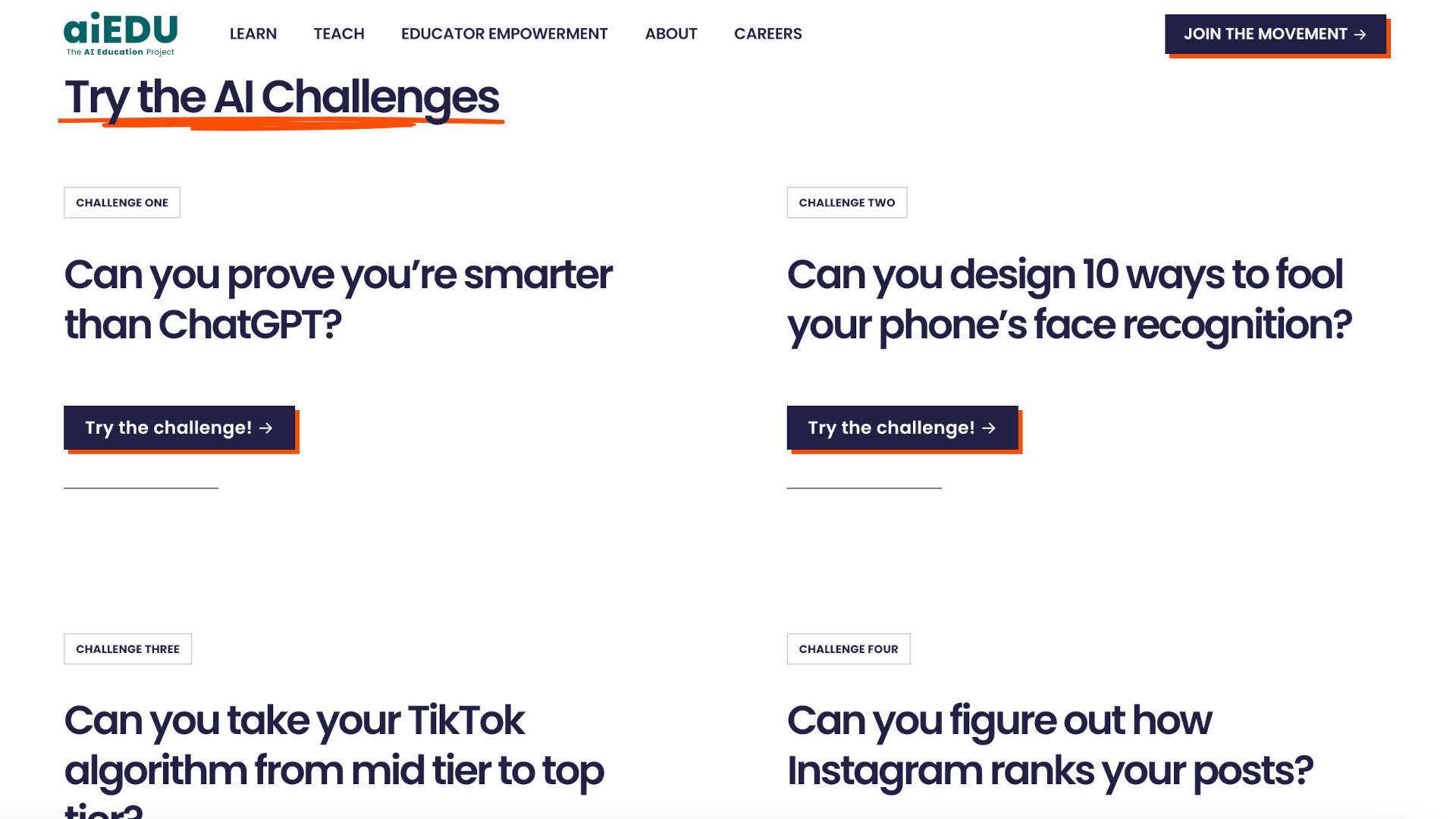The webpage titled "Try the AI Challenges" features a clean and modern design with a white background. In the upper left corner, the logo displays the text "AI, EDU" in a dark teal green, followed by smaller text reading "The AI Education Project." Beneath the logo, navigation options in black text are listed: "Learn and Teach," "Educator Empowerment," "About," and "Careers."

On the upper right corner, there is a prominent call-to-action button. The button is a long black rectangle underlined on the bottom and right side with an orange accent. It features white text that reads "Join the Movement."

Below this section, the page introduces several challenges. On the left side, there's a white rectangular box labeled "Challenge 1" in black text, followed by the prompt "Can You Prove You're Smarter Than Chat GPT?" Adjacent to it on the right side is "Challenge 2," asking, "Can You Design 10 Ways to Fool Your Phone's Face Recognition?" Each challenge is paired with a black rectangular button with orange underlining on the bottom and white text that says "Try the Challenge."

Further down, on the left, is "Challenge 3," which asks, "Can You Take Your TikTok Algorithm from Mid-Tier to Top Tier?" To the right, "Challenge 4" prompts, "Can You Figure Out How Instagram Ranks Your Posts?" Both of these challenges are also accompanied by black rectangular buttons with orange underlining on the bottom and white text that says "Try the Challenge."